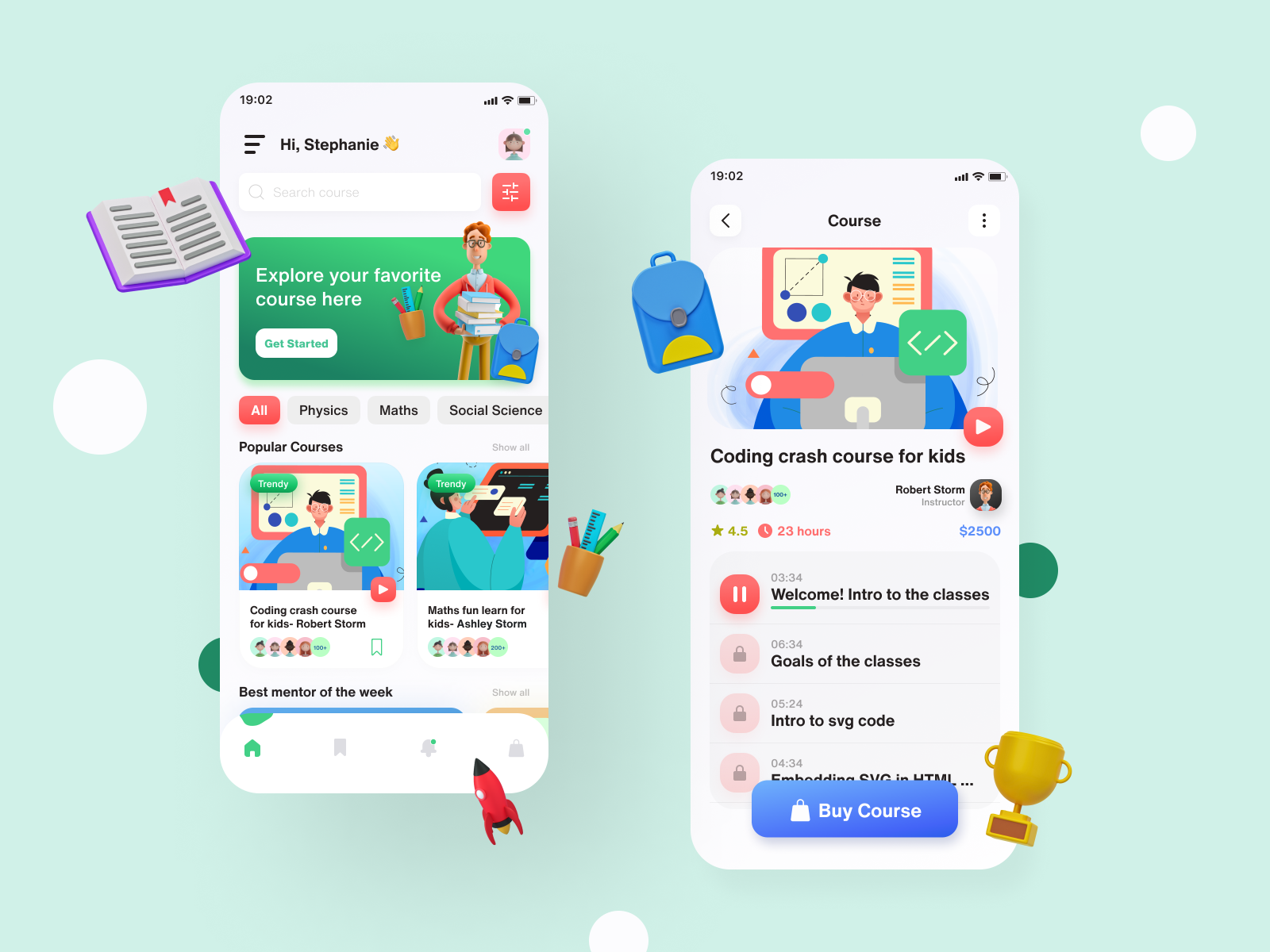This image serves as an advertisement for a course app, set against a light mint green background adorned with large white and darker green polka dots, giving it a playful and engaging appearance. At the center, two app screenshots are prominently displayed, with the left screenshot positioned slightly higher than the right.

The left screenshot depicts a mobile interface that greets the user, "Hi, Stephanie," accompanied by a waving hand icon. Beneath this, a search bar invites users to explore courses. A green button labeled "Explore your favorite course here. Get started" is present, surrounded by colorful, comic-style illustrations. Further down, there are various course categories listed: Physics, Maths, and Social Science. Additionally, specific course offerings such as "Coding Crash Course for Kids" and "Maths Fun Learn for Kids" are highlighted.

The right screenshot showcases another app screen titled "Course" at the top, featuring an animated person gazing at a computer screen. It promotes a "Coding Crash Course for Kids" priced at $2,500. Course details include "Welcome," "Intro to the class," "Goals of the classes," "Intro to SVG code," and another section partially obscured. At the bottom of this screen, a blue button prompts users to "Buy course."

Adjacent to these screenshots, whimsical comic-style illustrations of a book, a rocket ship, a trophy, and a backpack are scattered, enhancing the educational and adventurous feel of the advertisement.